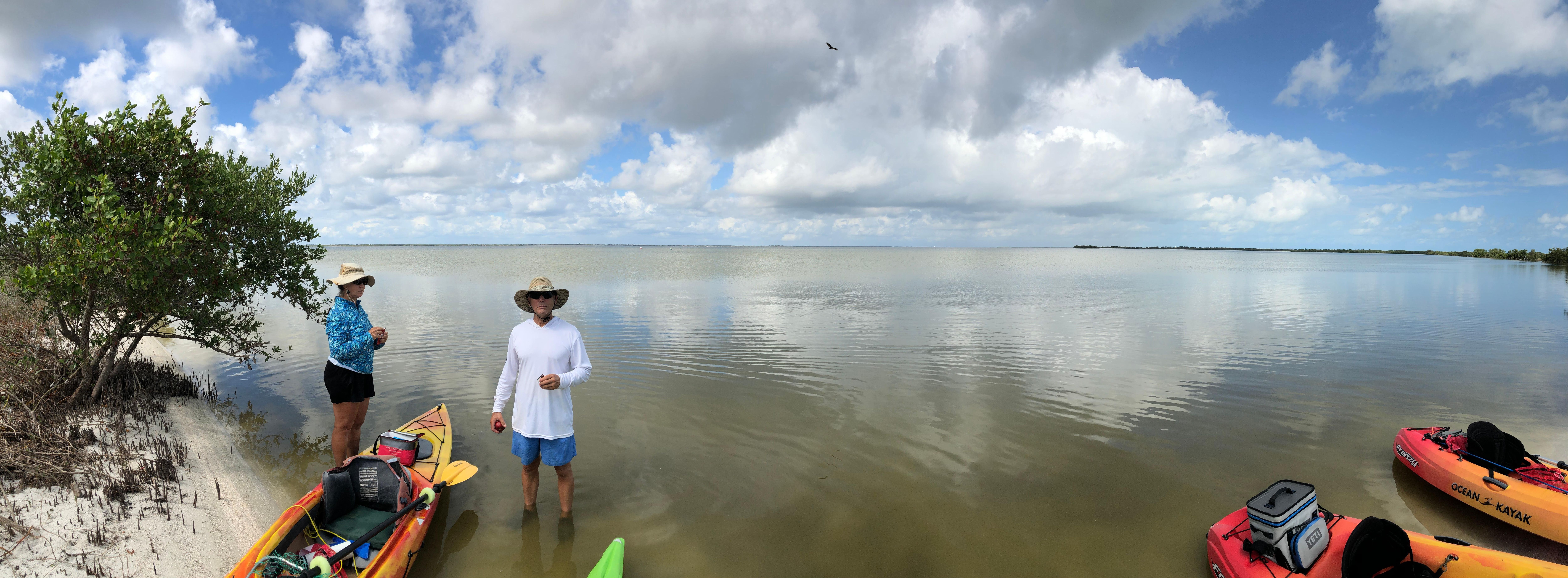In the panoramic outdoor shot of a serene lake with a murky blue-green hue, two individuals stand near the shore, immersed in a tranquil moment. The scene reveals a man and a woman, both adorned in sun hats and long-sleeved shirts for sun protection; the woman wears a beige hat, a blue top, and black shorts, while the man sports a beige hat, a white top, and light blue shorts. They're standing ankle-deep in the shallow water beside their reddish-orange kayak, appearing to take a break and maybe enjoying a snack, as the man gazes directly at the camera potentially holding an apple, and the woman looks off to the side introspectively.

The scene is dotted with a total of four kayaks: three clearly visible orange and reddish-pink ones and a partial glimpse of a green one at the bottom edge of the frame. Nearby, a couple of lunchboxes hint at a relaxing midday meal. A tree leans over the water from a small stretch of land on the left, providing natural shade. The sky further complements the scene with its bright blue expanse filled with fluffy white clouds, enhancing the scenic and peaceful outdoor ambiance.